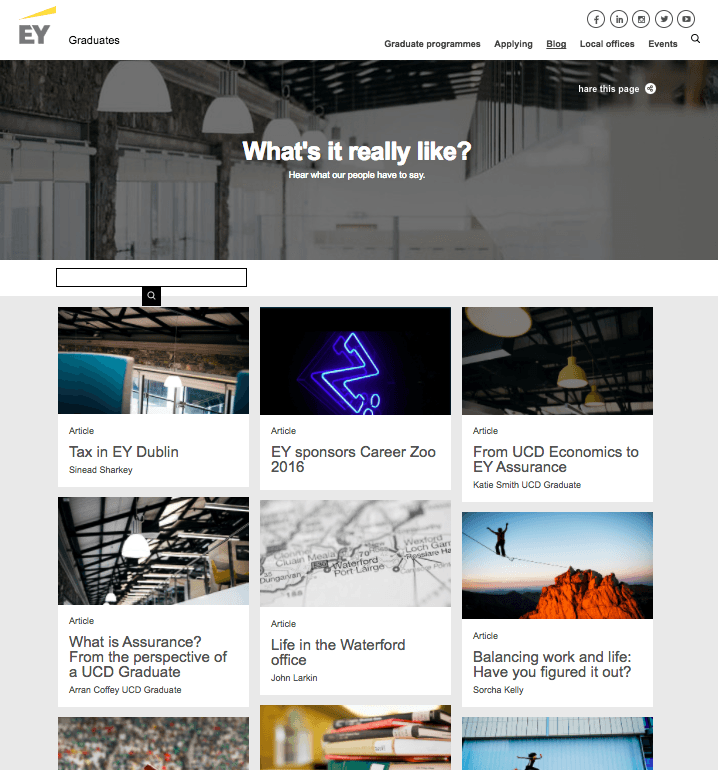The image is a detailed screenshot of a webpage, predominantly white in background. In the top left corner, the EY logo is displayed in gray letters, with a yellow triangle overhead. The word "graduates" is positioned next to the logo. To the right, the navigation menu includes the following options: "Graduate Programmes," "Applying," "Blog," "Local Offices," and "Events," indicating the use of British English as "programmes" is spelled with a double 'm' and 'e'.

Below the menu, a large, horizontally-aligned gray image is visible, depicting the interior of a room illuminated by numerous ceiling lights. The room has brown walls, and the entire image appears to be filtered in dark gray. Overlaid in white text are the questions: "What's it really like here? What do people have to say?"

Beneath this section, there is a grid of nine articles arranged in a 3x3 format. Each article is accompanied by a stock photo related to its content. The first six articles are fully visible, while only the images of the bottom three are partially discernible. The articles present the following headlines:

1. "Tax at EY Dublin, Shanice Starkey."
2. "EY Sponsors Career Zoo 2016."
3. "From UCD Economics to EY Assurance, Katie Smith, UCD Graduate."
4. "What is Assurance from the Perspective of a UCD Graduate, Aaron Coffey, UCD Graduate."
5. "Life in the Waterford Office, John Larkin."
6. "Balancing Work and Life, Have You Figured It Out?"

Each article features an image that visually represents the subject matter discussed in the accompanying text.